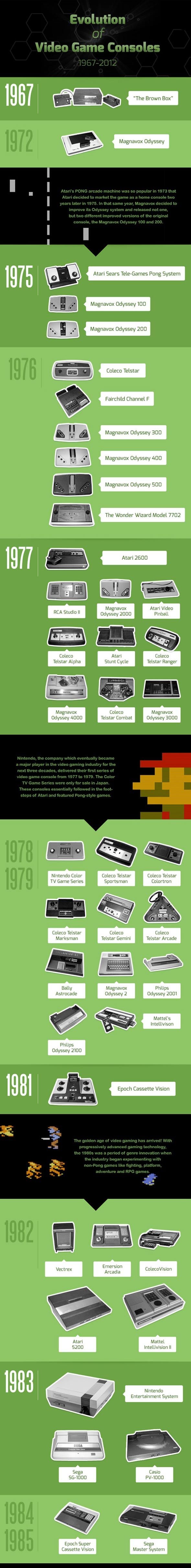The image is a vertically-oriented, detailed infographic titled "Evolution of Video Game Consoles 1967 to 2012," with a prominent black background at the top displaying the title in green text. The infographic is segmented into green and black horizontal strips, each representing different years and featuring small, indistinct images and conversation-like text boxes. Starting from 1967, it lists various iconic gaming consoles along a timeline, with each year neatly organized within its own green box. The image includes photos of the consoles, such as the Magnavox Odyssey, Atari's Pong, and Nintendo's early systems, alongside descriptive text bubbles providing historical context. Despite the low resolution and pixelated graphics, which make specific details hard to discern, the infographic visually narrates the chronological development of gaming hardware, marked by the introduction of each console from 1967 through 2012. Ascending text and small checkpoints within these horizontal segments underscore this progression, creating a structured, albeit lengthy, visual representation of gaming history.